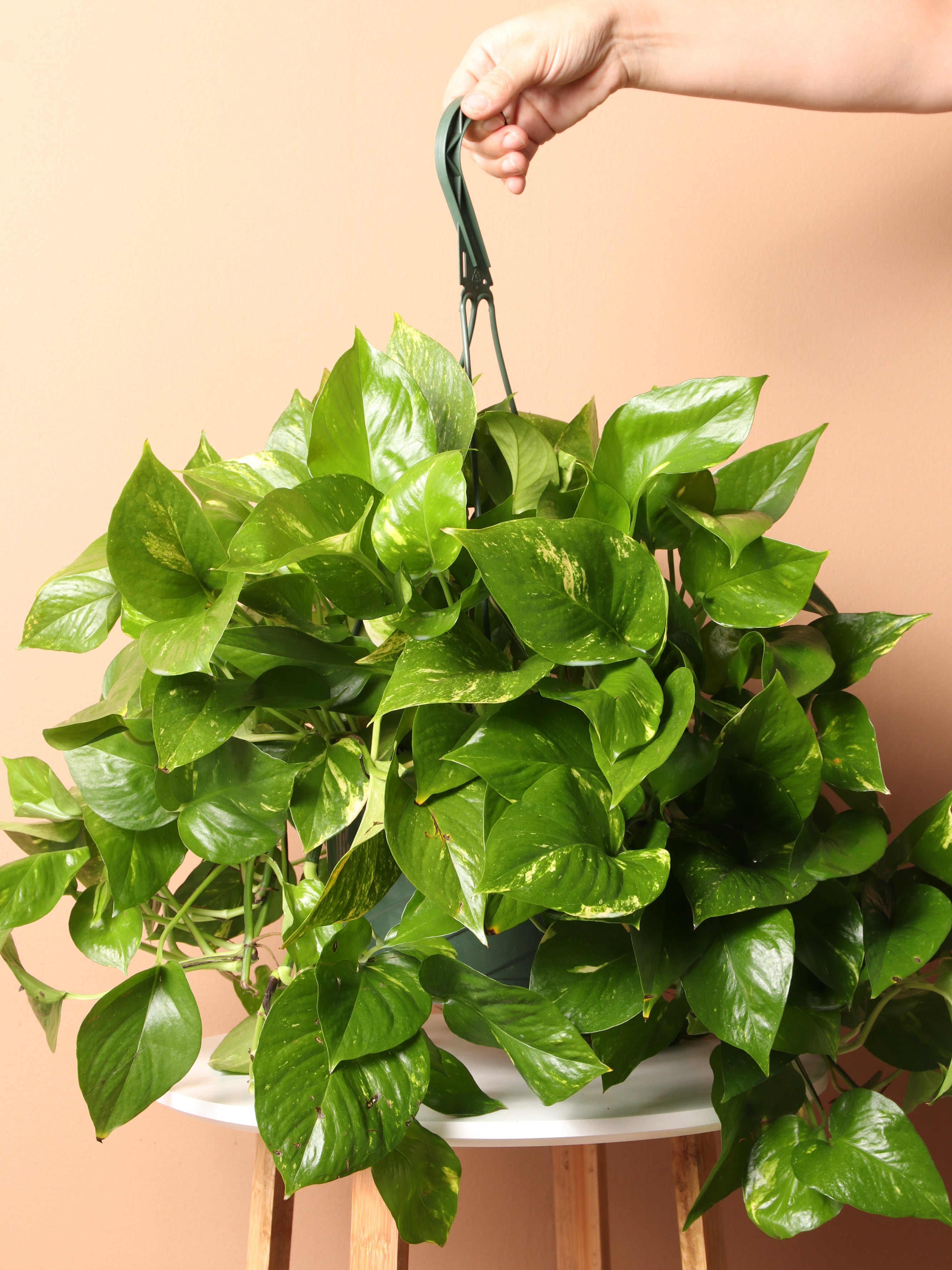In a well-lit portrait-oriented product photo, a vibrant, full, and healthy golden pothos, also known as devil's ivy, is prominently displayed against a light peach-colored background. The lush green leaves of the plant overflow and obscure much of the hanging pot, which is made of plastic and equipped with a green hook. The minimal browning at the ends of some leaves is barely noticeable. The plant, which is likely in a six to eight-inch pot, is being held by a hand extending from the top right corner of the image. Below the plant, a simple white tabletop with natural wooden legs, resembling a small white Ikea table or stool, is partially visible. The overall scene highlights the pothos's trailing vines and bright green, shiny leaves, dominating the photograph and giving it a very fresh and lively appearance.